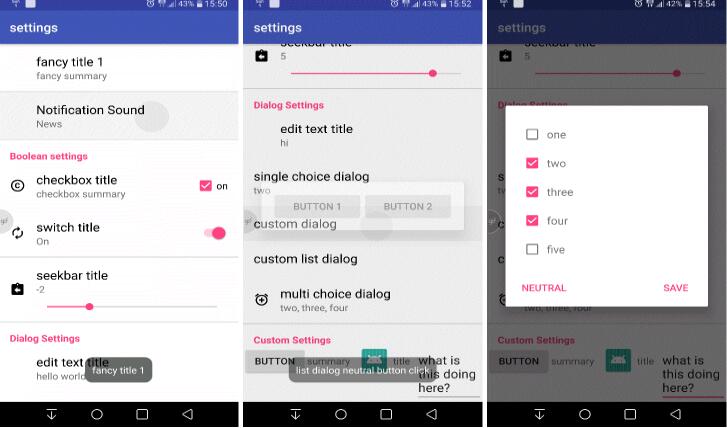The image is a composite of three separate screenshots from a device's settings interface, arranged to resemble a step-by-step instructional guide. 

1. **First Screenshot**: 
   - Title: "Fancy Title 1"
   - Instruction: Directs the user to navigate to "Notification Sound" within the settings menu.

2. **Second Screenshot**:
   - Instruction Continuation: 
     - Adjust the seek bar to level 5.
     - Modify dialog settings by changing:
       - Text title to "High"
       - Single choice dialog setting to "2"
       - Input custom dialog lists with multi-choice options set to "2, 3, and 4"
   - There is a button presented at the end to "Summarize" these changes.
   - Annotation: Contains a comment "What is this doing here?" referencing the list button.

3. **Third Screenshot**:
   - Displays an open white textbook-like interface with numbered items 1 through 5.
   - Items 1, 2, 3, and 4 are checked off with pink ticks inside white boxes, indicating selection.

This detailed and annotated visual guide illustrates various steps and settings adjustments, ultimately leading to checklist configurations as observed in the final part of the composite image.